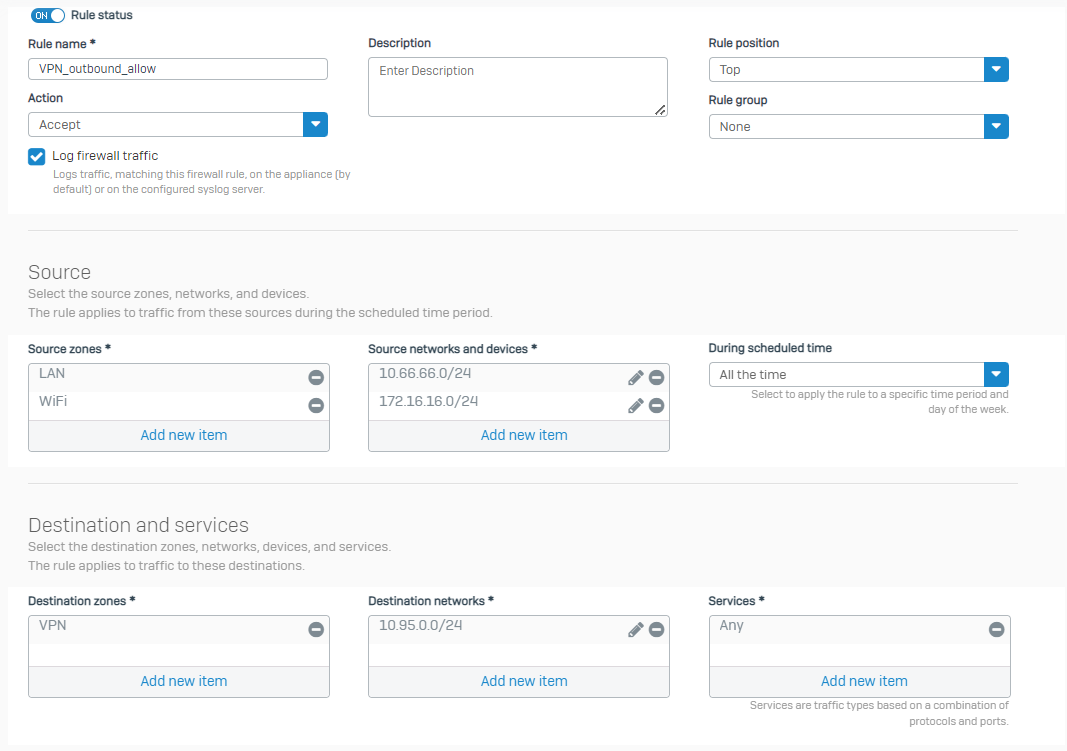The image depicts a web page interface designed for configuring security rules, most likely associated with a file-sharing platform or security suite. The interface features a clean white background with predominantly black text. 

At the very top left corner, there is a label "Rule Status" accompanied by a toggle switch that can be turned on. Below this, there is a section titled "Rule Name" with the current rule named "VPN_outbound_allow." Directly beneath this section is an "Action" field set to "Accept," which can be changed via a drop-down menu.

To the right, there is a "Description" field inviting the user to "Enter description." Adjacent to this is the "Rule Position" field set to "Top," also with a drop-down menu. Additionally, there is a "Rule Group" field with a drop-down menu for selection.

Further down, the option to "Log Firewall Traffic" is available. The following sections pertain to source and destination configurations. The "Source" section instructs the user to select source zones, networks, and devices, clarifying that the rule applies to traffic from these sources during the scheduled time period. The destination configuration fields similarly include "Destination Zones," "Destination Networks," and "Services."